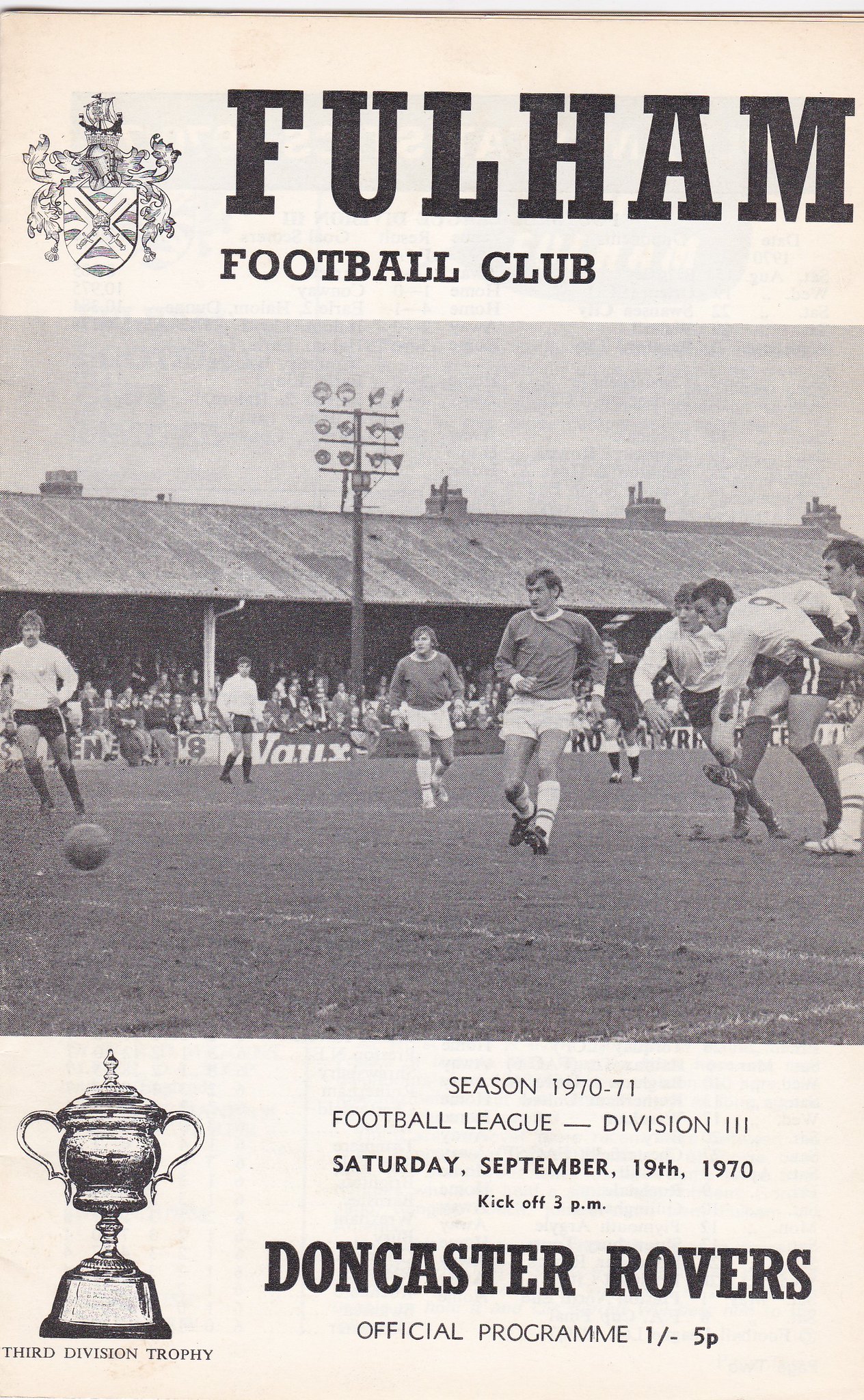The image depicts a vintage football program cover from the Fulham Football Club, dated Saturday, September 19, 1970. The title "FULHAM FOOTBALL CLUB" is prominently displayed at the top in bold black letters on an aged, beige paper background. An emblem or heraldry shield is noticeable on the top left. Below the title, detailed text reveals the season information, stating "Season 1970-71 Football League Division Three." The central part of the cover features a stark black and white photograph capturing a lively soccer match with players in contrasting uniforms – darker jerseys with white shorts versus white jerseys with darker shorts – all vying for the ball amidst a backdrop of numerous spectators seated under covered stands, with large arena lights visible overhead. Towards the bottom, on the left side, there is an illustration of a trophy labeled "Third Division Trophy," and to the right, the text "Doncaster Rovers Official Program" alongside the price "One Per 5 Pence" is printed. The overall design indicates that this program was a purchasable item providing essential details and schedules for the match day.